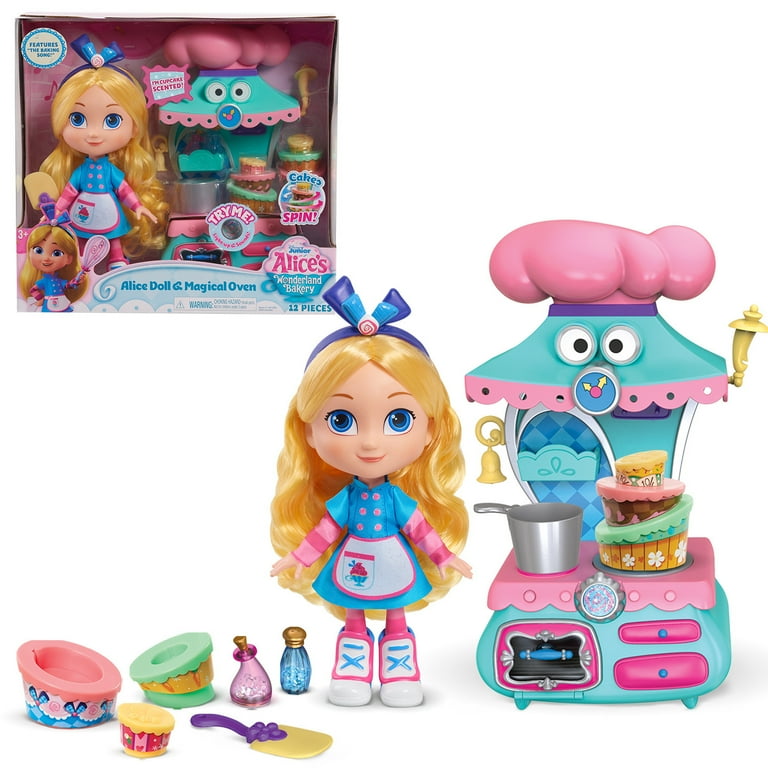This image showcases an Alice's Wonderland Bakery toy playset, designed for children, featuring a detailed and imaginative kitchen setup alongside a doll. The playset is presented against a plain white background, with the top left corner depicting the original packaging—a square cardboard and plastic box. The box prominently displays the name "Alice doll and magical oven" and various other descriptions, and illustrations of the contents. 

Inside the set, there is a blonde Alice doll with big blue eyes, adorned in a blue and pink dress, a pink and gray apron with designs, and white and pink shoes with blue laces. She also has a purple and blue bow tied at the back of her hair. Beside her stands a whimsical oven creature, colored blue and pink, complete with white and black eyes, a chef's hat, and a nose that resembles a clock. The oven features two pink drawers and a teal and pink body.

Accompanying these main items are several baking accessories: a yellow spatula with a purple handle, a pan situated on one of the oven's burners, a three-layer cake, a cupcake, salt and pepper shakers, and various small green, pink, and red-orange utensils and accessories. The oven also includes a pot and a bell. 

Together, these pieces invite imaginative play, allowing children to recreate baking adventures straight out of Alice's Wonderland Bakery.